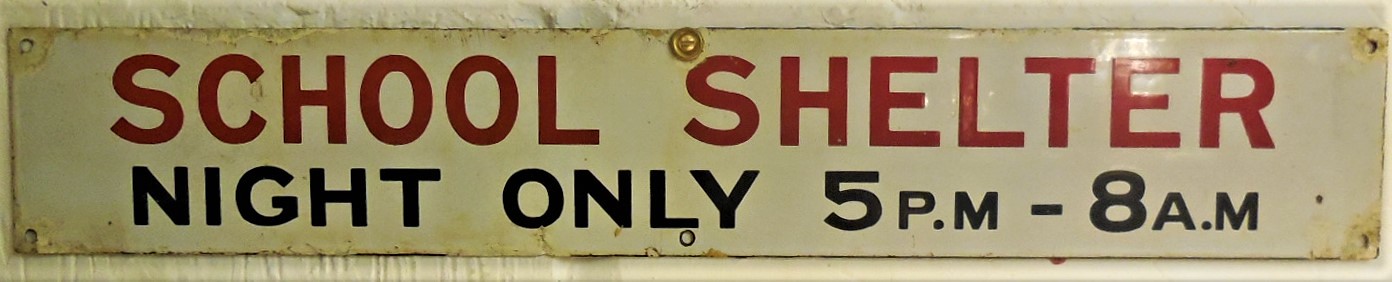This photograph features a long, narrow, metal sign mounted on a textured white wall, secured by a single nail or screw at the top center. The sign, which shows signs of aging with rust, yellowing, and browning around the nail holes and edges, reads "SCHOOL SHELTER" in large red capital letters. Beneath that, in black text, it states "NIGHT ONLY, 5 PM to 8 AM." The sign also has three nail holes each at the top and bottom edges, positioned at the left, right, and center, though only the top center one remains in use. This sign likely denotes a designated shelter area operational during nighttime hours, possibly for wartime, tornado safety, or other emergency situations.